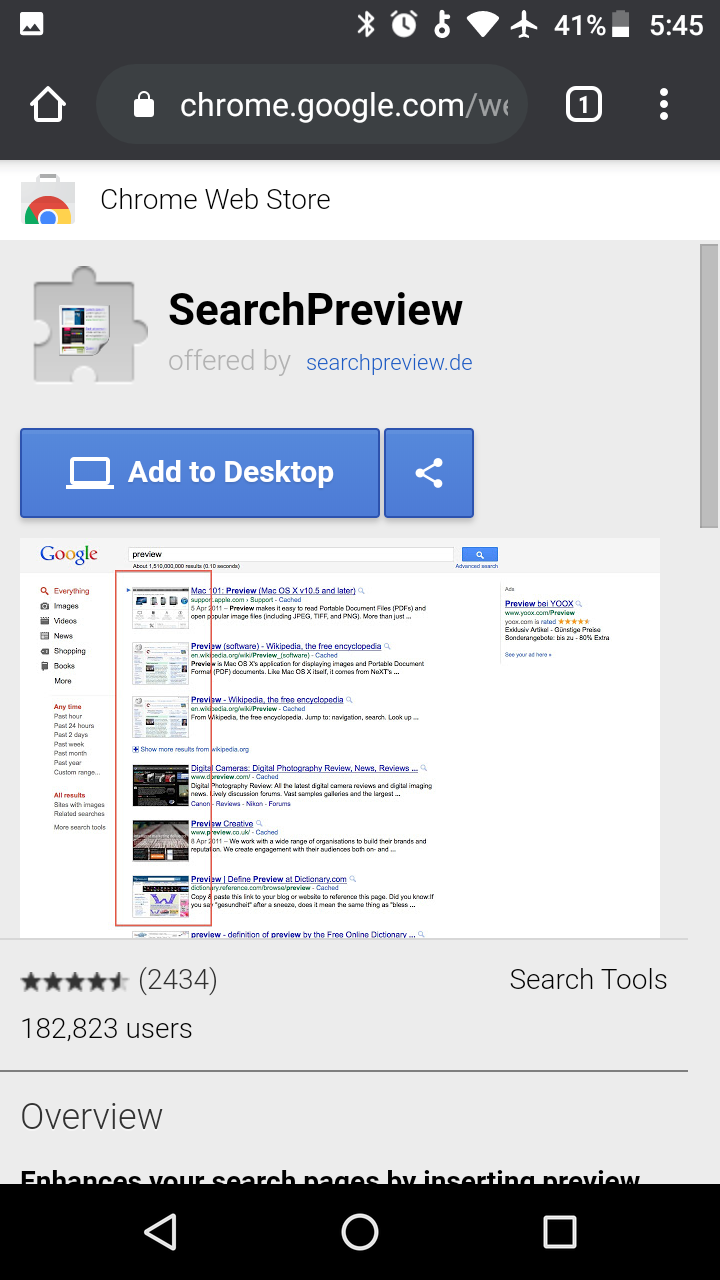The image depicts an unreleased app named "Search Preview," identified by its interface and the label "search preview offered by search preview.de." The user interface has a prominent button labeled "Add to Desktop" with an option to share, allowing others to download it. Below this, there's a feature allowing previews of search results similar to Google Search, marked by boxes outlining various websites. The app has an impressive user engagement with 182,000 users and corresponding ratings, although specific details on ratings are not provided. A partially visible "Overview" section indicates that the app enhances the search page by inserting previews.

Navigational elements include a back button, an exit button (indicated by a circle), and a search bar at the top, suitable for integration with Chrome. The browser shows only one open tab, and the device is noted to be in airplane mode. Additional device details include a battery level at 41% and the time reading 5:45 PM. This app appears to be in an experimental phase, potentially available for testing before its public release.